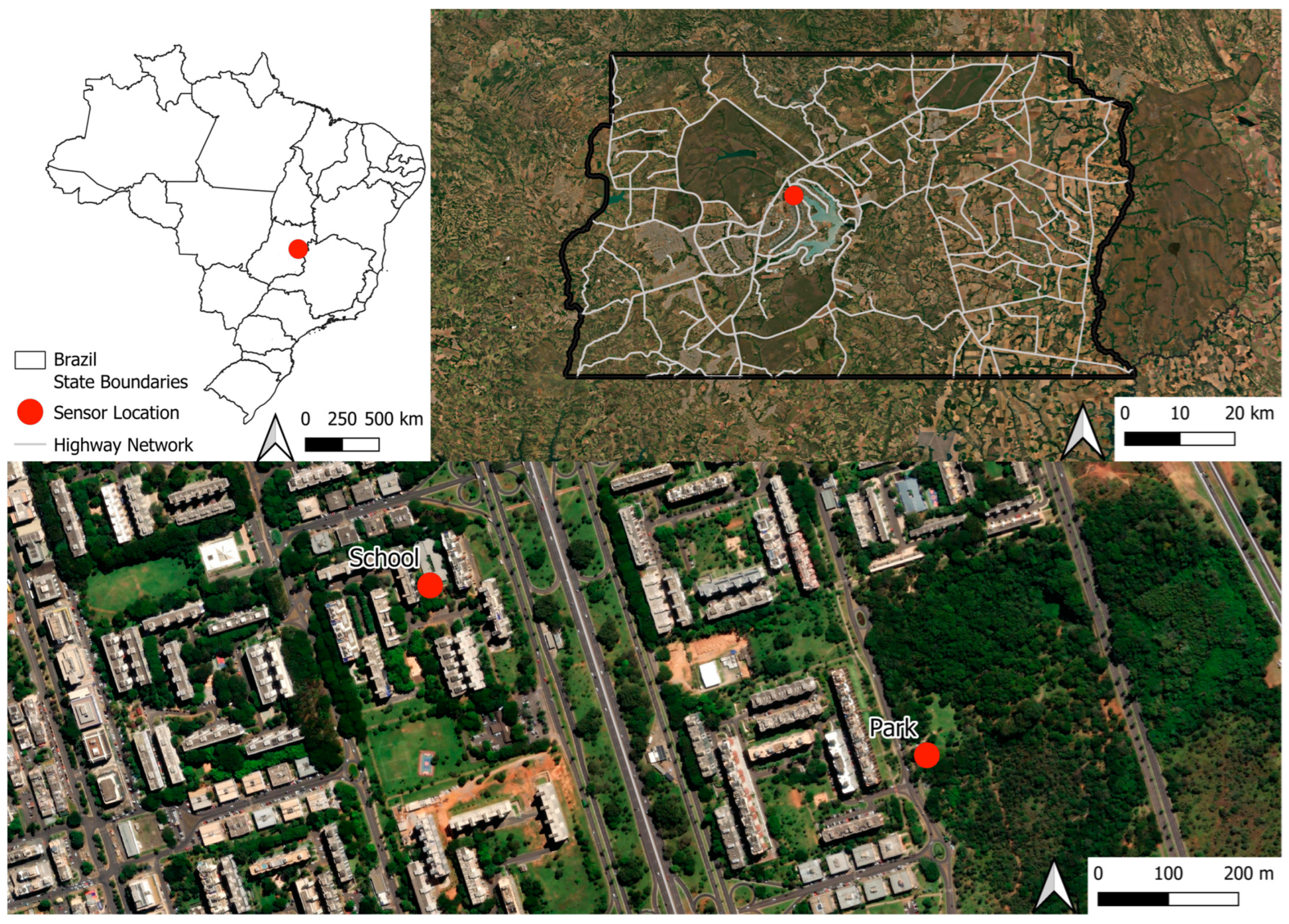The image is a detailed composite map with three distinct sections. The main section at the bottom displays an aerial photograph of a neighborhood, showcasing a bustling landscape filled with houses, buildings, roads, and lush green areas. Clearly marked with red dots are two important locations: a "school" towards the middle and a "park" in the lower left-hand corner. The area brims with trees, providing a vivid sense of greenery. A scale indicating distances of 0, 100, and 200 meters can be found in the bottom right corner of this aerial view.

Above this aerial photograph are two additional maps. The map on the left is a computer-generated graphic illustrating Brazil's state boundaries, identified by a rectangular outline, highway networks depicted with lines, and a sensor location marked with a red circle. This map includes a scale bar showing distances of 0, 250, and 500 kilometers. To the right, a satellite-style map provides a closer, detailed view of the landscape with roads marked in white and another key area marked by a red circle. This map also features a scale, indicating distances of 0, 10, and 20 kilometers.

Overall, these three sections together provide a rich and layered understanding of the area, presenting both macro and micro perspectives through detailed annotations and clear, informative legends.